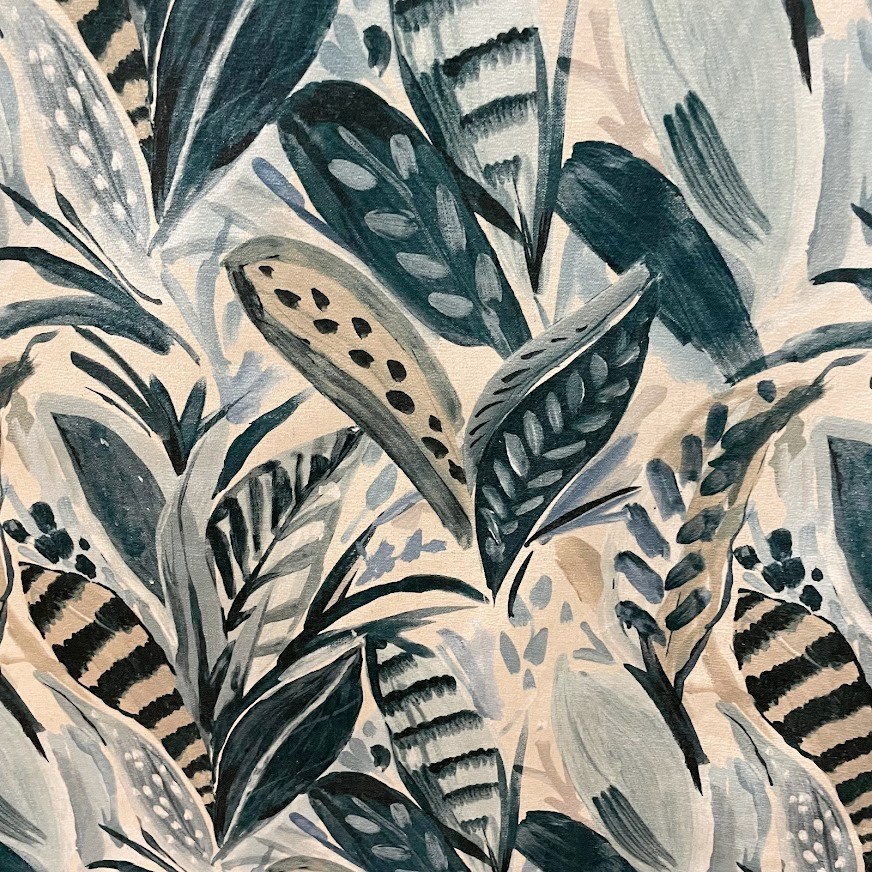A delicate watercolor painting captures a myriad of elongated fern and plant leaves intricately interwoven across a muted beige background that almost resembles a soft khaki or light pink shade. The artwork showcases an impressive array of around 20 to 30 distinct leaves, each characterized by varying subtle hues and patterns. Among them, there are leaves adorned with black polka dots elongated into oval shapes, and others featuring white oval-shaped specks. Some leaves present unique stripe patterns akin to zebra or tiger tails, in a subdued palette of black, brown, and gray, while others exhibit a bluish-green tint with white specks. Additionally, there are tan leaves with black specks outlined by dark gray borders. Amidst this harmonious tangle, some leaves stand out in solid dark colors or feature bean-like shapes along their sides. Notably, the absence of stems, trunks, or roots shifts the focus entirely on the delicate and diverse foliage, each element reaching upward and contributing to the intricate, layered composition of this understated and elegant painting.